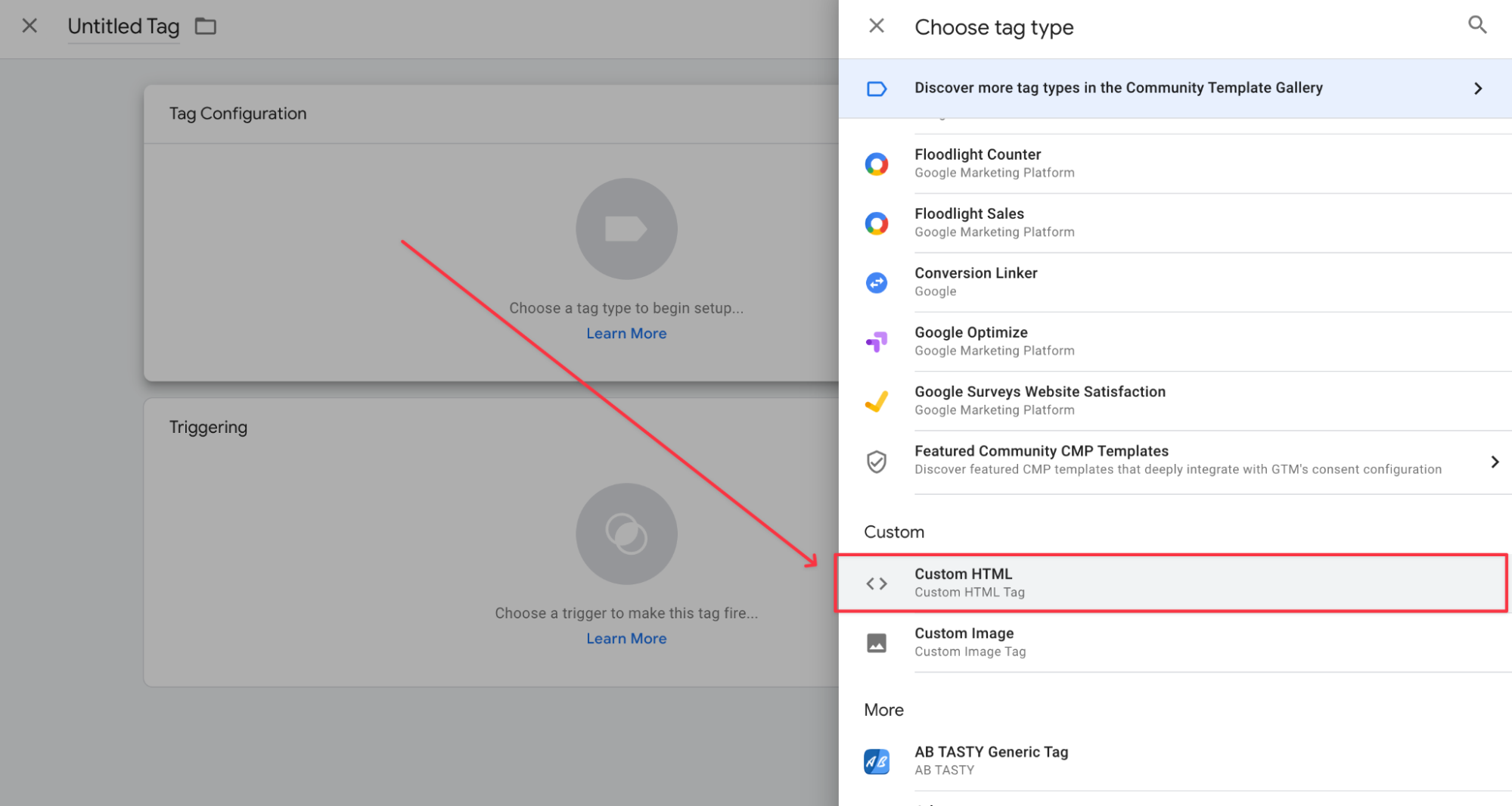This image showcases a user interface of a marketing or advertising platform, likely a Google-related tool, displaying a pop-out menu on the right-hand side. The menu's header reads "Choose tag type," followed by a list of tagging options available to the user. These options include "Floodlight Counter," "Floodlight Sales," "Conversion Linker," "Google Optimize," "Google Surveys," "Website Satisfaction," "Featured Community CMP Templates," "Custom HTML," and "Custom Image." There is also a "More" section that includes "A/B Tasty" and "Generic Tag."

Highlighted within the menu, with a red border and a long arrow pointing to it, is the "Custom HTML" option, drawing attention to this specific tag type. Beneath the main list, there is a prompt to "Discover more tag types in the community template gallery" with an accompanying link.

The majority of the interface outside this menu is a gray area labeled "Tag Configuration and Triggering," which appears to be empty. This layout suggests the user is in the process of configuring a custom HTML tag, with the highlighted element indicating a focal point for additional inputs or configurations.